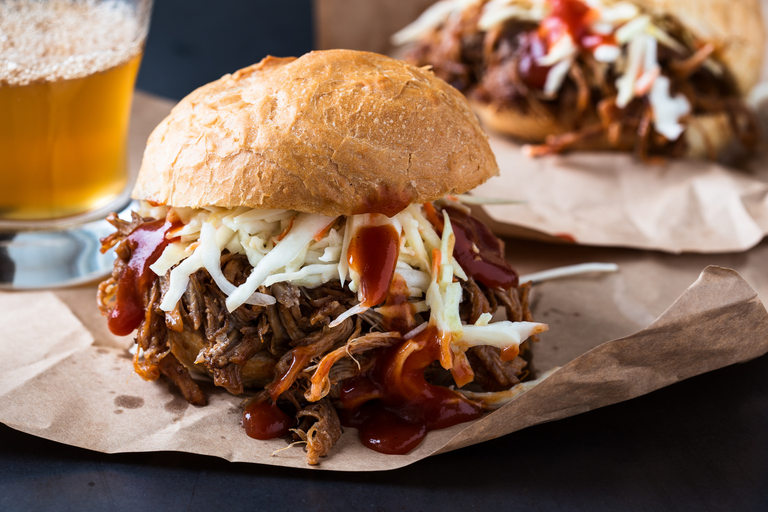This image is a close-up photograph featuring a pulled pork barbecue sandwich prominently in the center, resting on a piece of crumpled brown paper placed on a dark gray tabletop. The sandwich is messily constructed with a dome-shaped brown bun on top. Beneath the bun, there are shredded white cheese or coleslaw strands visible, topped with a generous amount of brown barbecue sauce that drips down onto the brown paper. The pulled pork beneath the sauce appears thick and stringy, piled high within the sandwich. In the upper left corner of the photo, there is a glass filled about a third of the way with a yellowish liquid, presumably beer, exhibiting a foamy top. The upper right background shows another sandwich, slightly out of focus, suggesting a similar pulled pork item but with the top bun dislodged. The overall color palette includes shades of brown, white, yellow, gray, and hints of red from the barbecue sauce. No words or text are present in the image.